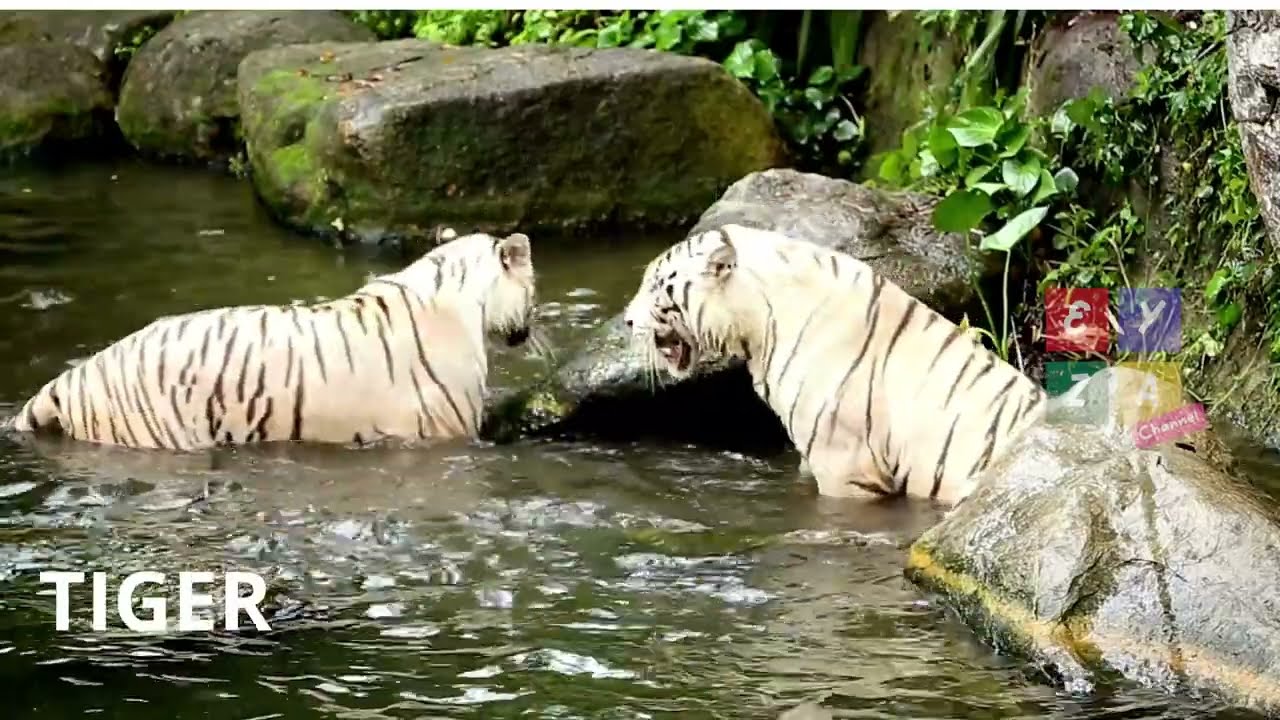The image depicts two white tigers with black stripes standing in murky, greenish-brown water, likely within a controlled environment such as a zoo. Large gray stones and boulders, some covered with moss and algae, frame the scene. The left tiger, facing away from the camera but looking back towards the right, contrasts with the right tiger, which is facing the left with its mouth open, displaying sharp bottom teeth. A tall, rock wall covered in green foliage and plants forms the background on the right. In the lower left corner of the image, the word "TIGER" is clearly written in white text. On the right-hand side, the letters "E Y Z A" appear in colorful boxes—red for E, blue for Y, green for Z, and yellow for A—with a small pink box diagonally below these letters.